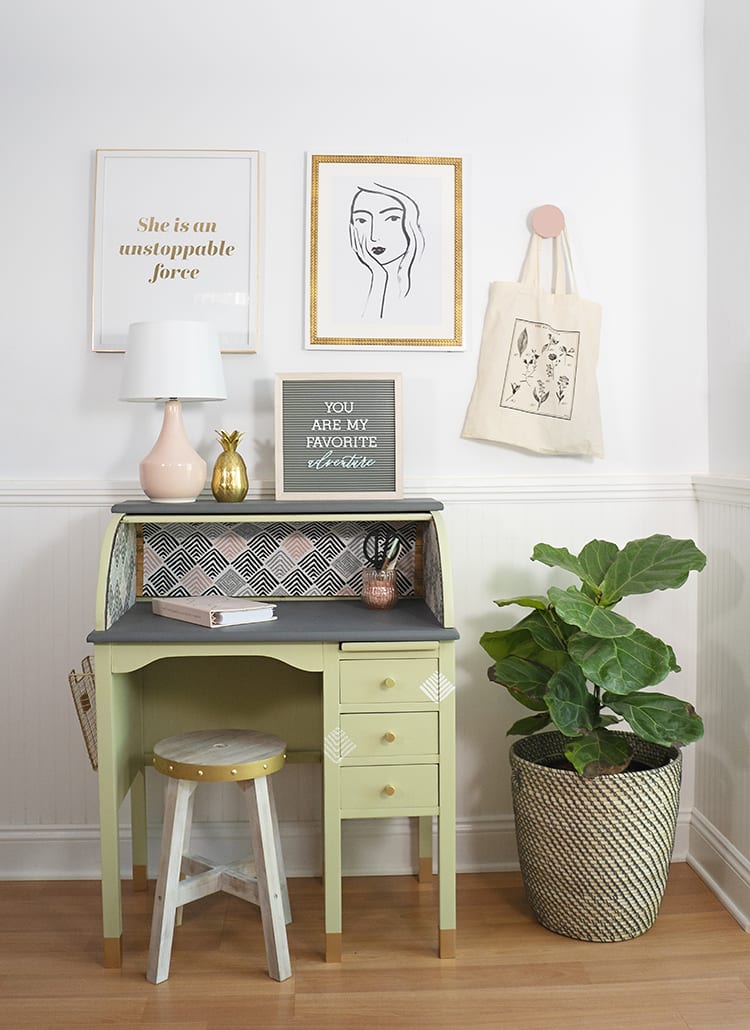This indoor bedroom image showcases a thoughtfully arranged, feminine-designed space. Central to the scene is a small lime green desk, adorned with a subtle pattern and accompanied by a white painted wooden stool featuring a circular seat. On the desk sits a pink lamp, a gold pineapple-shaped decoration, and a gray-colored book. Additionally, a cup holds various office supplies, including scissors and pencils. The desk also features three drawers positioned on the right side.

Above the desk, a sign with cursive lettering reads, "You are my favorite..." though the last word remains unclear. To the left, another sign, in white with gold letters, declares, "She is an unstoppable force." Below this sign and to the right hangs a pencil sketch of a woman's face, her right hand gently touching her cheek, gazing outward. Further contributing to the room's décor, a canvas tote bag is suspended on the right side of the wall.

In the corner, a large green-leaved plant stands about 2 to 3 feet tall, nestled in a stylish gold and black pot on an elevated plant stand. The room's white walls, complemented by wainscoting, and laminated brown wooden floor create a balanced backdrop for this chic and motivational setup.